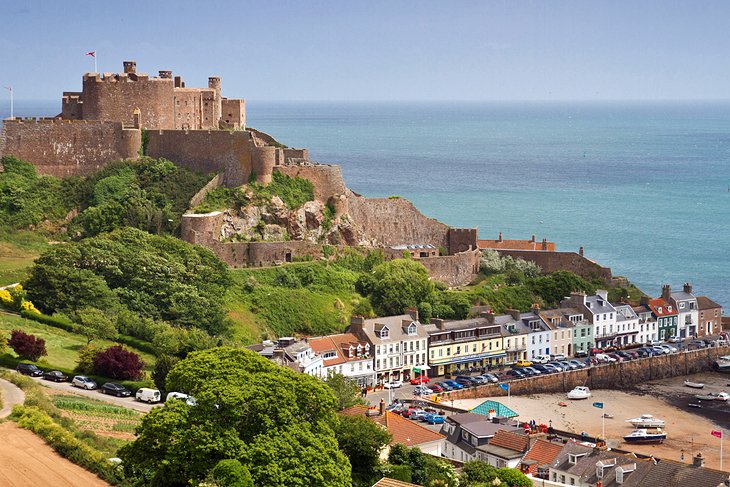The image captures a picturesque, daytime scene featuring a vibrant blue sky and an expansive blue ocean stretching into the distance. In the upper left corner stands a grand, brown castle adorned with red flags, perched majestically atop a hillside. The hillside itself is part of a bustling city or town, where winding roads at the base of the hill are lined with an array of parked vehicles, including white vans and SUVs. The area is lush with greenery, as clusters of trees with dense foliage dot the landscape. The scene also showcases rolling hills that gently slope towards clusters of buildings. These buildings consist of approximately 35 attached houses in various colors, creating a charming patchwork effect. Near the shore, a serene beach is seen with boats anchored peacefully. The entire setting encapsulates a harmonious blend of natural beauty and urban life, all under the bright, clear sunlight.